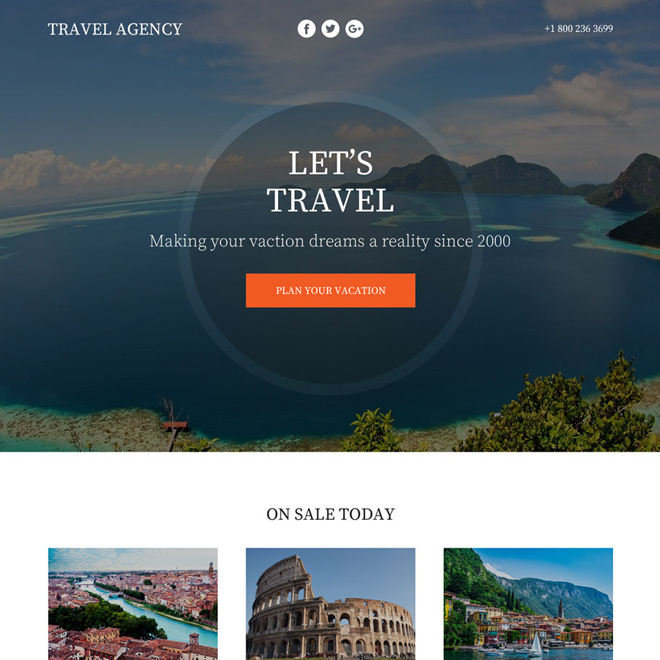A captivating travel agency advertisement showcases a tranquil tropical landscape. At the forefront, a vast, serene blue lake is the centerpiece, bordered by small patches of lush land on the upper left and right. Majestic mountains rise on the right side, under a sky painted in brilliant blue and adorned with scattered white clouds. The foreground in the bottom right is dotted with vibrant green shrubs, adding to the idyllic scene.

Prominently displayed in the center of the image is the inviting text: "Let's Travel - Making Your Vacation Dreams a Reality Since 2000." Below this enticing statement, an eye-catching orange button reads "Plan Your Vacation."

In the top left corner, the travel agency's name is elegantly inscribed in white, while the top right features social media icons for Facebook, Twitter, and Google, along with a contact phone number. The lower section of the advertisement showcases three enticing images labeled "On Sale Today," highlighting various picturesque destinations available at special rates, beckoning travelers to embark on their next memorable adventure.